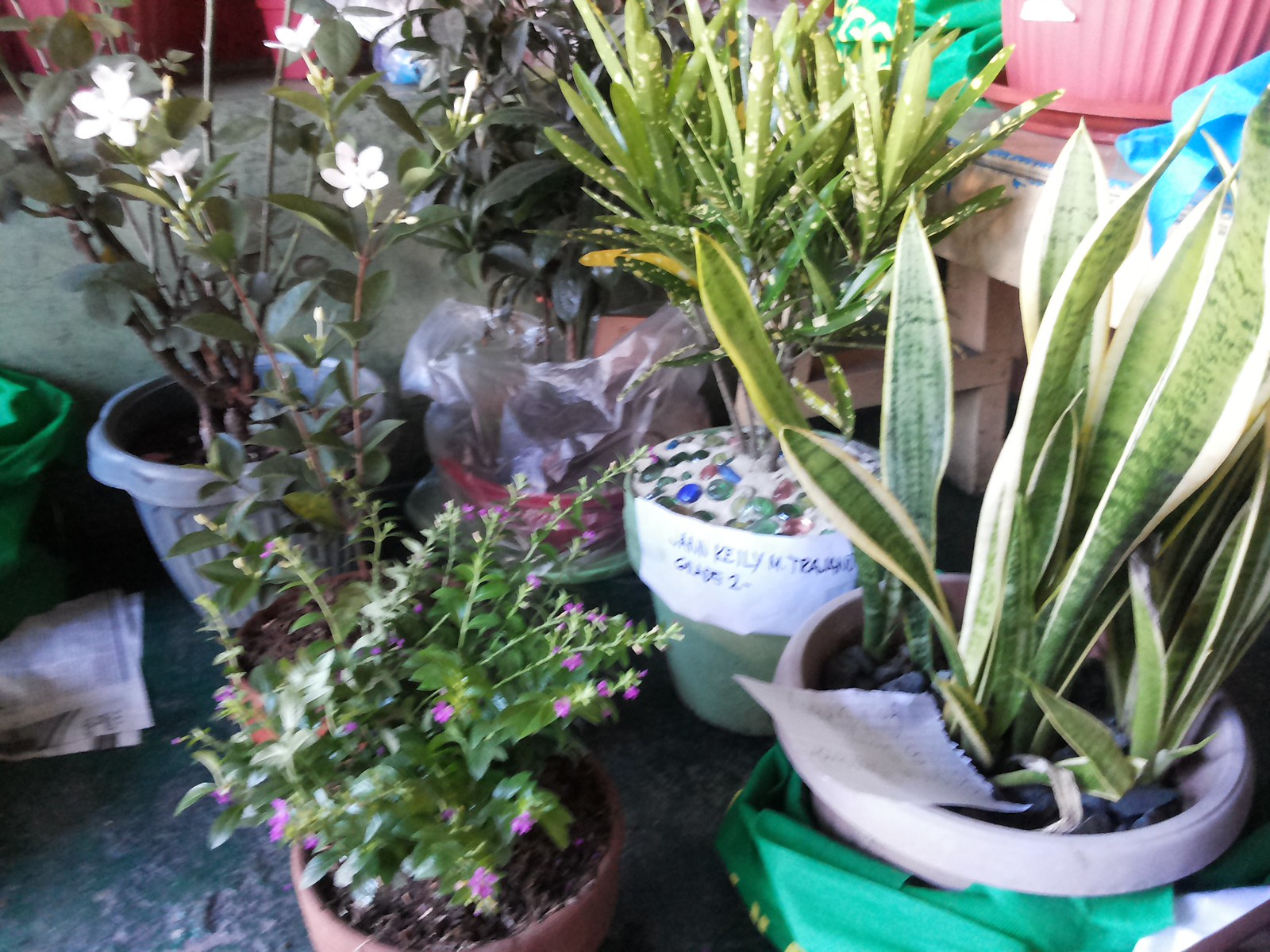The photograph captures a diverse assembly of potted houseplants arranged on what seems to be a back porch area. The floor, a green-painted but chipped cement surface, is scattered with newspapers and empty potting soil bags. Center stage are approximately seven to eight main houseplants, each in varying pots—ranging from ceramic to plastic and even nestled inside reusable green bags. The pots themselves are a mix of colors like pink, gray, and tan, adding eclectic charm.

Among the plants, there's a notable variety: a variegated snake plant with long, green leaves bordered in white sits prominently on the far right. Another pot features a tall, viney plant with white flowers blooming at the top, while a different container holds a small, bushy plant adorned with tiny purple flowers. Additionally, some plants have broad green leaves, enhancing the visual texture. In the back, resting on a wooden workbench, is another potted plant which adds depth to the composition.

All these elements combine to make a lush, lived-in botanical corner, brimming with life and color, encapsulated in this detailed snapshot of someone's gardening haven.